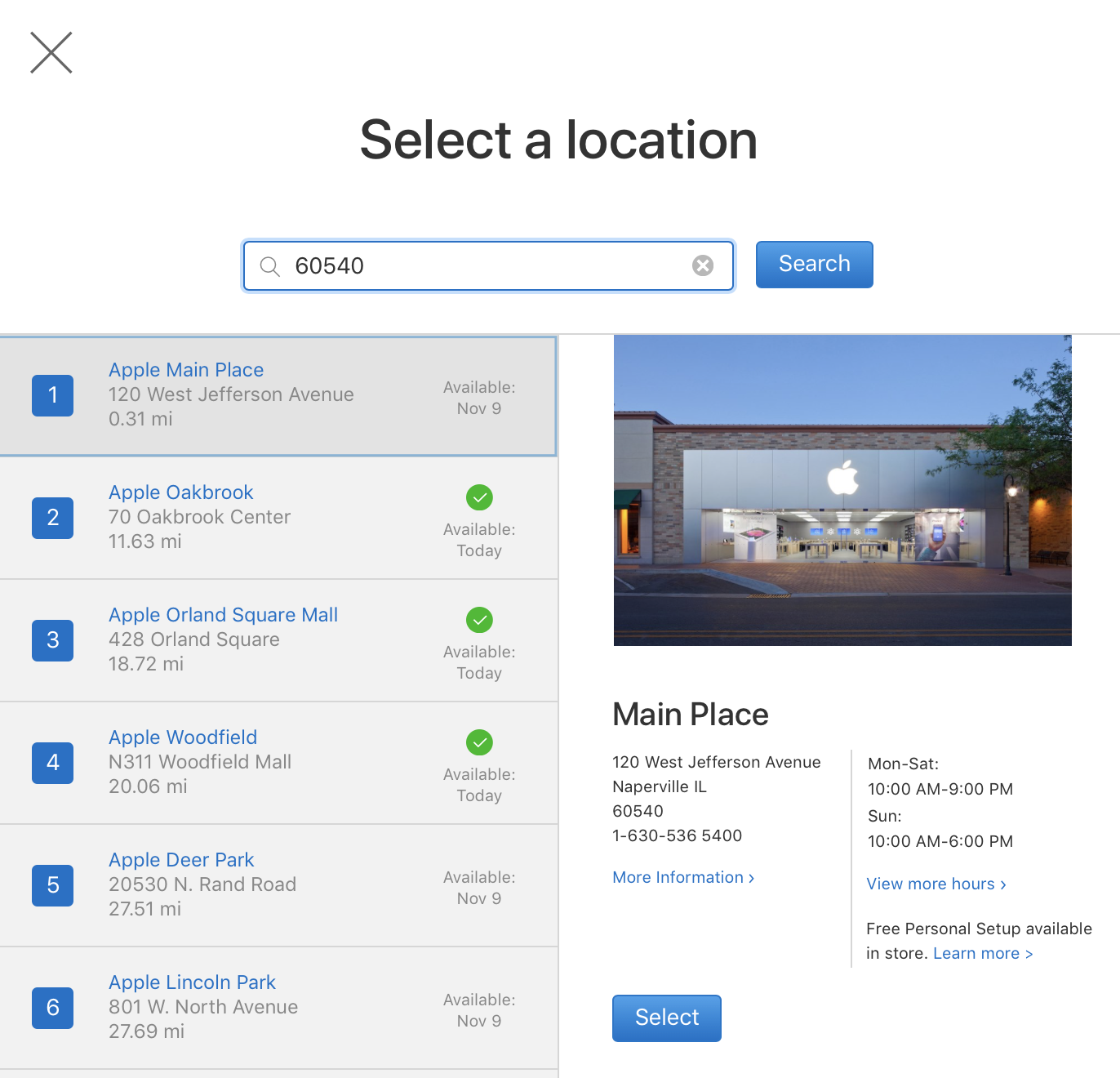The image features a web interface for selecting an Apple Store location. At the top, bold black text reads "Select a Location." Below it, a white search box framed by a blue line, set against a white background, invites the user to enter a zip code. Upon entering, the interface displays six Apple Store options, indicating availability for appointments or services:

1. **Apple Main Place** in Naperville, available starting November 9th.
2. **Apple Oak Brook**, available today.
3. **Apple Orland Square Mall**, available today.
4. **Apple Woodfield**, available today.
5. **Apple Deer Park**, available starting November 9th.
6. **Apple Lincoln Park**, available starting November 9th.

The Apple Main Place store in Naperville is highlighted, showing its operating hours: 10 AM to 9 PM, Monday through Saturday, and 10 AM to 6 PM on Sunday. The overall scene suggests the user is looking to book an appointment or visit an Apple Store, with a specific emphasis on the Naperville location.